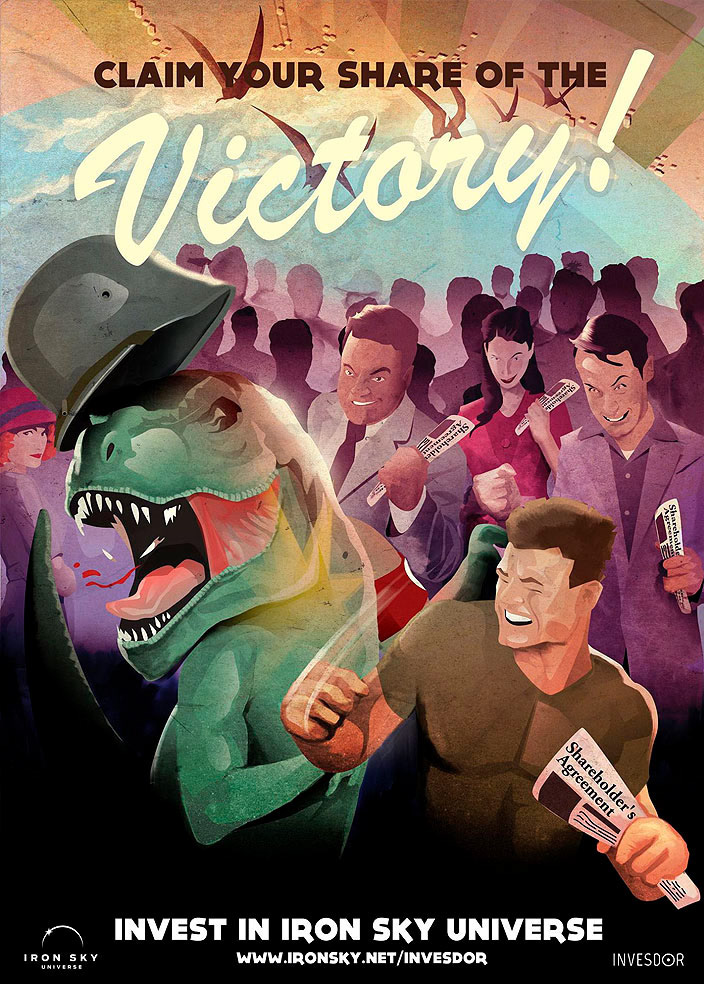The image appears to be an advertisement poster, possibly for a movie or a magazine cover, showcasing an eclectic and vibrant scene. The background transitions from green and white stripes to a blue circular shape, adorned with brown birds flying across the top. Prominently, the top of the image features the phrase "Claim Your Share of the Victory!" in large, casual white cursive letters. Below, a diverse crowd of people is depicted. In the distance, the people are mere silhouettes, while the foreground reveals detailed characters: a woman in a red dress holding a rolled-up paper, two men in gray suits also clutching papers, and a green T-Rex wearing a black military hat. The T-Rex is being punched in the face by a man wearing an army fatigue t-shirt, with teeth flying out of its mouth. Behind the dinosaur stands a woman with crossed arms, donning a red and blue hat and sporting orange hair. In a blacked-out area below, the words "Orange Sky Universe" appear alongside a half-circle logo, emphasizing an investment opportunity with the text "Invest in Orange Sky Universe, www.orangesky.net/invesdor." The newspaper held by several characters prominently displays "Shareholders Agreement," and the corner of the image features "Invesdor" in small white letters. The overall palette of the image incorporates purples and blues, adding to its dramatic and eye-catching appeal.